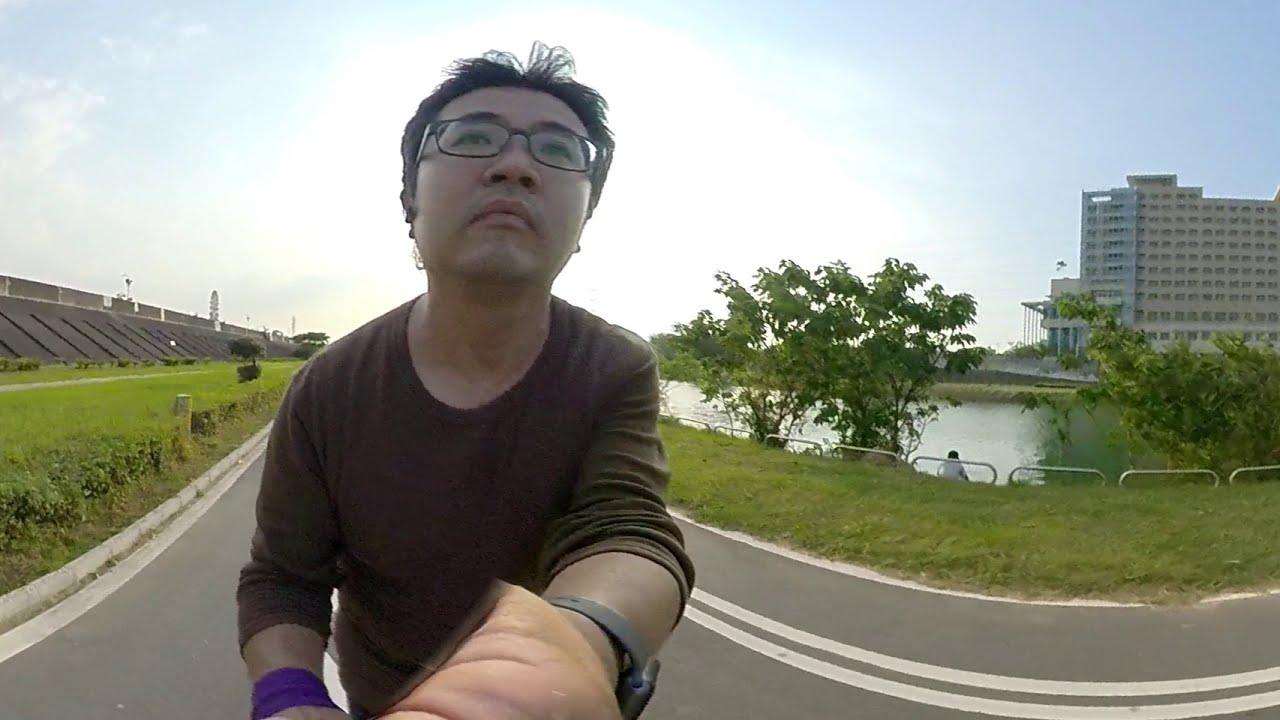The image depicts an Oriental man, appearing to be in his 20s, positioned slightly to the left of center on a dark gray, paved street with a white double line running across it. He is possibly riding a bike, though only visible from the waist up, giving the impression he is high off the ground. The man has short black hair, wears glasses, a brown long-sleeved shirt, a wristwatch on his left wrist, a purple wristband on his right wrist, and possibly a glove on his left hand. He is looking slightly upwards towards the vivid blue sky, with the sun seemingly behind his head. The street curves to the right behind him. To his right, there is a grassy area followed by a large gray office building with numerous windows, trees, and a pond where someone in a white shirt is sitting on the bank. To his left, the street is bordered by grass and a cement hill that looks like an elevated highway structure, with what appears to be bleachers midway up.